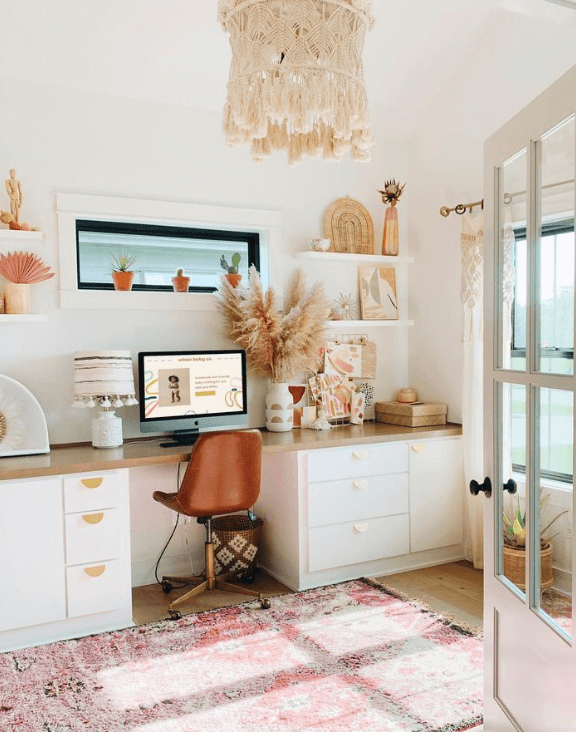The image showcases a small, light-filled home office space with a predominantly white color scheme, giving it a bright and airy feel. The main focal point is a long white desk aligned against the back wall, supporting a large computer monitor. In front of the desk sits a brown-backed, wheeled chair. The desk features three narrow drawers on the left and three wider drawers on the right, alongside a small cabinet. 

Above the desk, there are several white shelves adorned with various decorations, including a small golden statue, a vase filled with what appears to be pink peacock feathers, and a butterfly painting. A mix of potted cacti in reddish clay pots adds a touch of greenery to the scene. 

Adjacent to the desk is a window, accompanied by another larger window on the right side, both allowing ample daylight into the room. This right window is framed by a light pink curtain pulled to the left. Below this window, there is a potted plant and an open door with four clear glass panes and a black circular doorknob. The wooden floor is partially covered by a multicolored pink, white, and black area rug with intricate embroidered designs. 

Overall, the decor includes subtle salmon or pink-colored accents, such as a white and off-pink desk lamp and various decorations on the shelves, contributing to the room's cozy and inviting atmosphere.